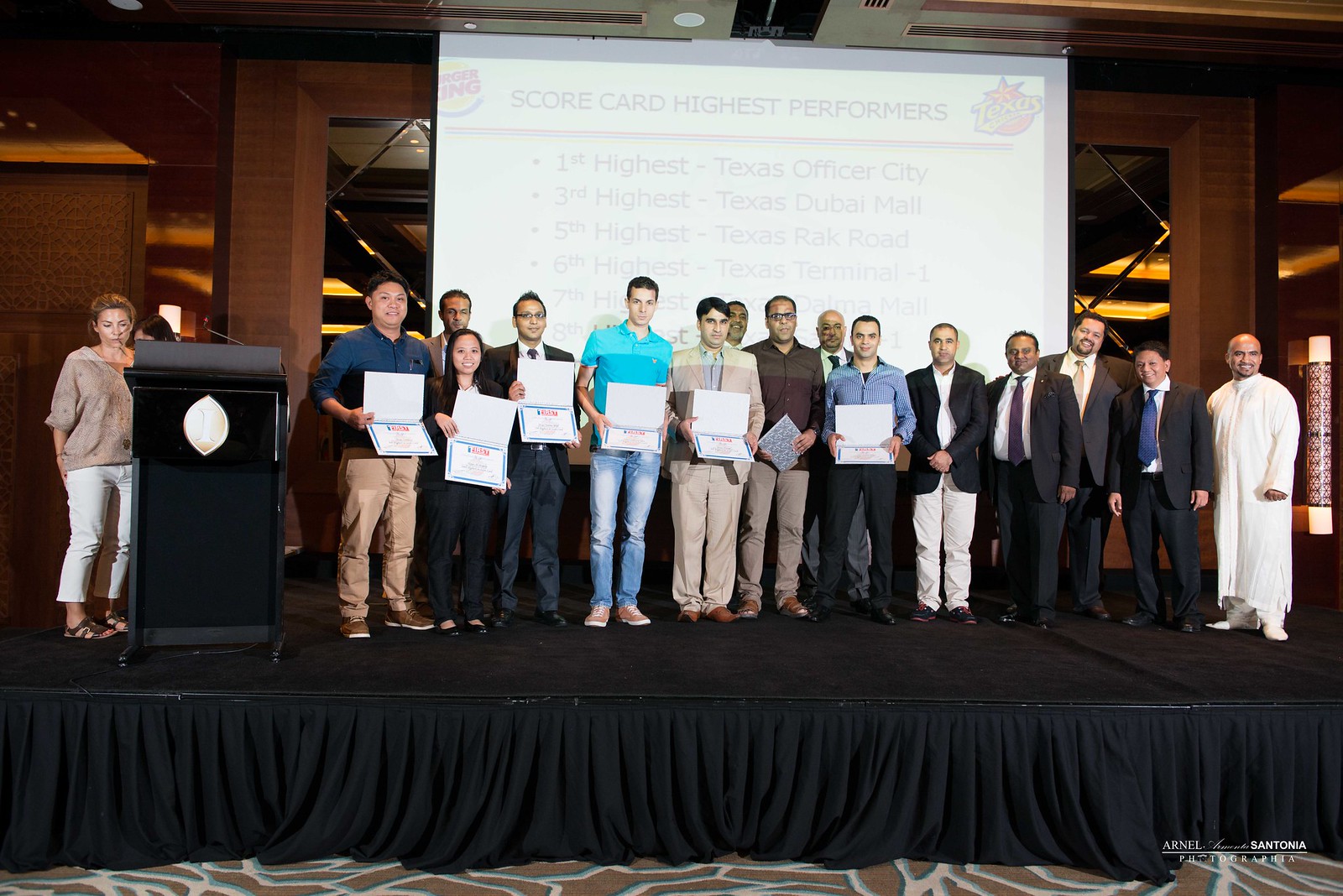The photograph captures a group of 16 people standing in a horizontal line on an elevated black stage, which features a black curtain around its base. They are mostly men, with at least two women among them, and are dressed in a mix of formal and casual attire, including suits, collared shirts, and even blue jeans. Among them, a man in religious attire is positioned on the far right, wearing a white robe and gold iconography around his neck. A woman is stationed behind a podium on the left, possibly aiding as an event coordinator.

Behind them, a large, white screen with a gray frame displays a PowerPoint presentation. On the top left, a Burger King symbol is visible, while the right corner features a Texas-related logo. The title on the screen reads "Scorecard: Highest Performers," listing rankings such as "1st: Texas Officer City," "3rd: Texas Dubai Mall," "5th: Texas Rack Road," and "6th: Texas Terminal One," with some additional faded listings obscured by the group.

The stage is set within a large, high-ceilinged room with red walls and reddish-brown pillars flanking the screen. The floor in front of the stage has a brown and white carpet. Various members hold certificates or awards, posing with them prominently for the photograph, indicating their recognition as highest performers.